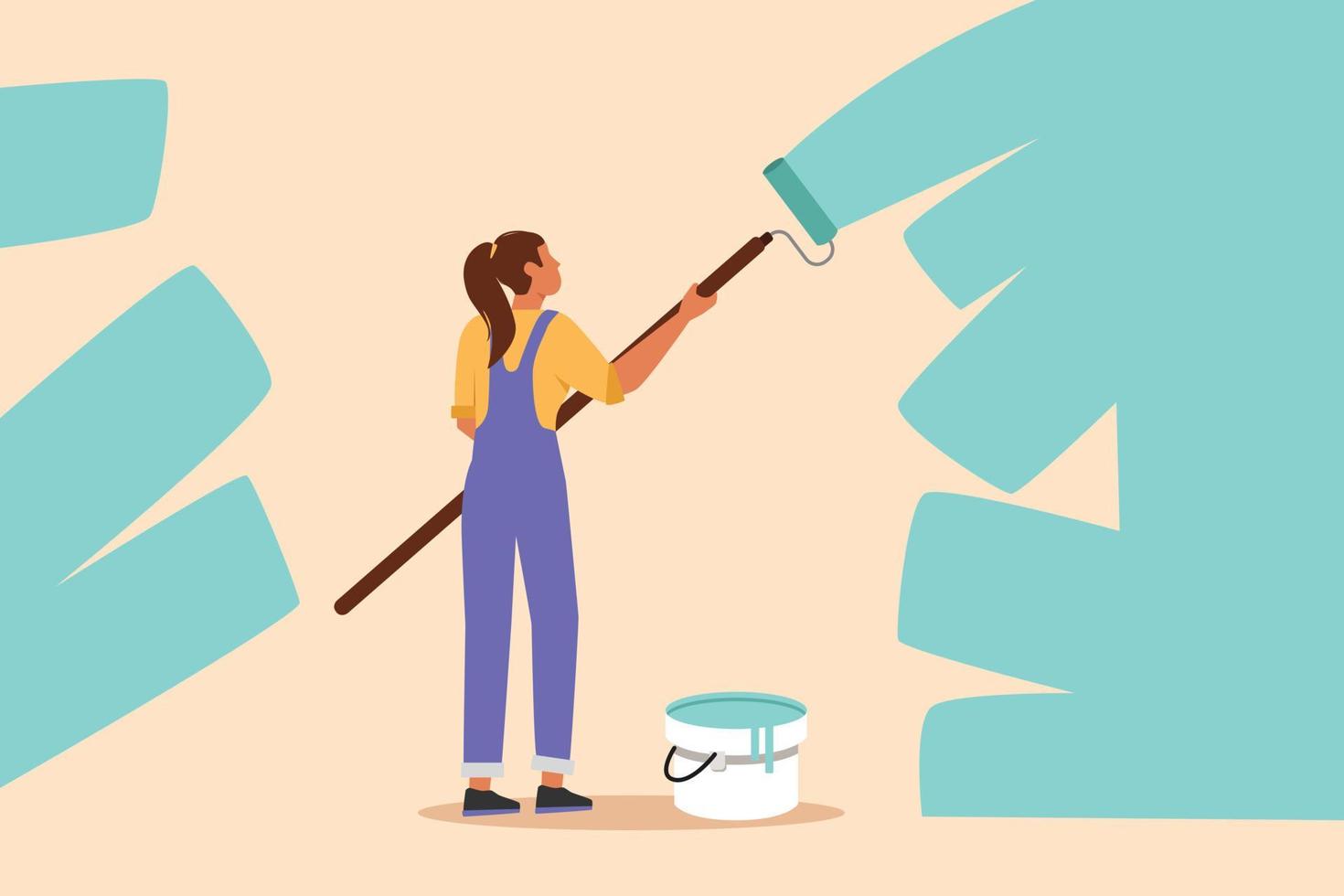This digital graphic depicts a female cartoon character engaged in painting a wall. Positioned slightly off-center but primarily in the middle of the image, the woman stands with her back to the viewer, holding a long-handled paint roller in her hand, which is raised towards the upper right. She is at the early stages of the painting process, some sections of the wall showing a greenish-peach base color, while other parts have been covered in fresh teal paint. 

The character has light brown skin, long brown hair, and wears a yellow long-sleeve top beneath a purple overall, accented by a blue outer layer. On the floor to her right, there is a white bucket filled with blue paint. The setting is simple with no text or additional elements, emphasizing the act of painting itself. The color palette includes tones of purple, yellow, brown, tan, teal, bluish-green, black, and white, which contribute to the overall warm and creative ambiance of the scene.